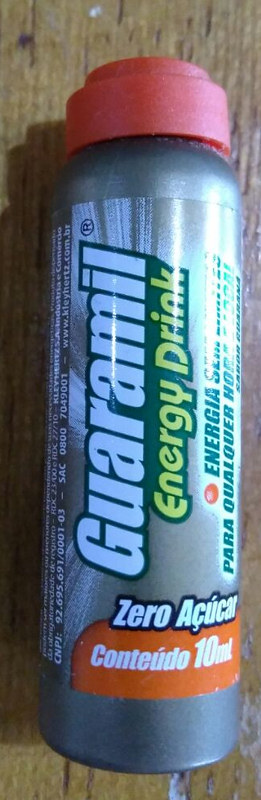This close-up color photograph features a metallic grey, cylindrical bottle of Guaramil Energy Drink, occupying 90% of the image and set against a wooden background. The bottle, which can be easily mistaken for a can due to its material, has a striking red cap. The labeling is predominantly in Spanish or Portuguese, with "Guaramil Energy Drink, Energia" written horizontally in white. The text "zero azúcar," meaning "zero sugar," is also visible, alongside "Contende 10 mil," all in white lettering. The bottle's design incorporates vibrant yellow, green, and orange hues, with green text detailing additional information. The image is well-lit, with a pronounced light source from the right side causing a bright strip that washes out parts of the logo, casting a shadow to the left of the bottle.